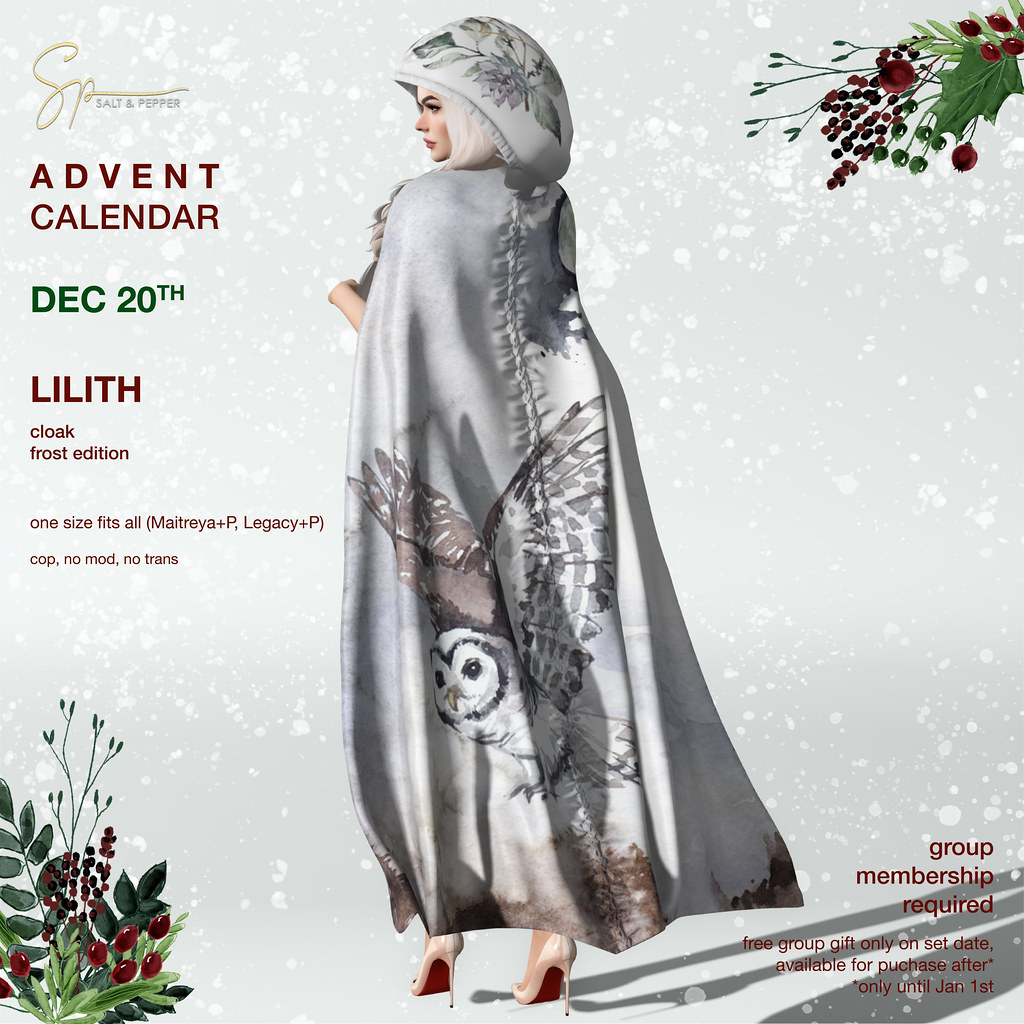The digital event poster features a cartoon image of a woman with her back to the viewers, standing center stage. She is adorned in a long, flowing, hooded robe that is gray in color and detailed with a striking design of an owl in flight. Her white hair cascades to her right, partially visible. She steps elegantly in cream-colored stiletto heels with red soles. Snow is gently falling around her, evoking a serene winter scene, enhanced by decorative holly and plants situated in the bottom left and top right corners against a predominantly white background.

In the top left corner, the logo "SP" appears with the text "Salt and Pepper" below it. Adjacent, the text reads: "Advent Calendar December 20th" in red and green fonts. Further detailed information is listed as "Lilith Cloak Frost Edition," and notes the cloak as "One Size Fits All" with sizing compatibility denoted as "(Maitreya + P, Legacy + P)." The terms "Cop, No Mod, No Trans" are included, indicating the item's usage restrictions.

At the bottom right corner, red text specifies "Group Membership Required. Free Group Gift Only on Set Date. Available for Purchase After Only Until Jan 1st." The overall ambiance of the poster highlights the exclusivity and limited availability of the "Lilith Cloak Frost Edition," showcased in a festive and wintry aesthetic.